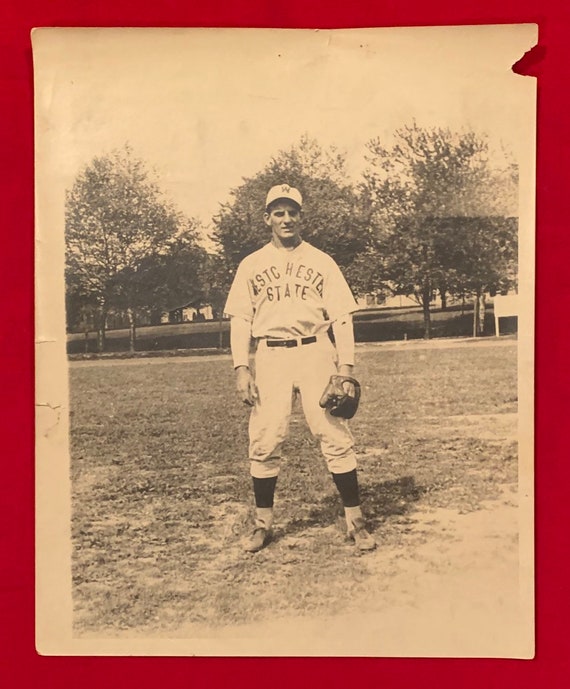The weathered black-and-white photograph, now faded to a sepia tone, captures a baseball player standing in a grassy field. The man is dressed in a vintage baseball uniform, consisting of white capri-style pants, black socks, a short-sleeved jersey over a long-sleeved undershirt, and a black belt. His uniform features partial letters on the front, including “E-S-T-C-H-E-S-T” and “S-T-A-T-E,” partially obscured. He wears a white cap marked with the letter "W" and holds a baseball glove on his left hand. The background reveals patches of dirt amidst the grass and a line of large trees against the bright sky. The edges of the photo are worn, with a small tear at the top right corner and a white border framing the image, which sits on a red background.